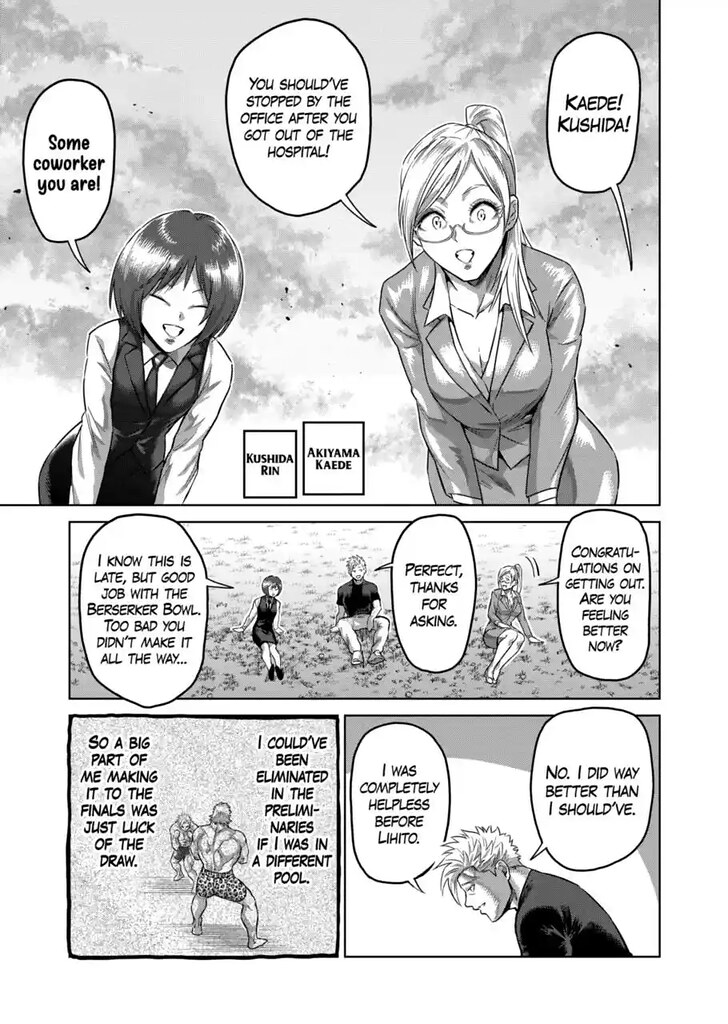The black and white comic strip features four panels in a vertical rectangle format, with a background in shades of gray. The top panel, spanning the full width, depicts two women in conversation, both bending towards the viewer. The woman on the left, Kushida Rin, has short brown hair, wears a white long-sleeve shirt with a tie and a vest, and smiles with her eyes closed. She laughingly says, "Some co-worker you are." The woman on the right, Akiyama Cade, taller with long blonde hair partly in a ponytail, glasses, and a professional suit that shows some cleavage, replies, "You should have stopped by the office after you got out of the hospital."

In the second, central panel, the same two women and a man with blonde spiky hair are seated on the grass. Kushida Rin says, "I know this is late, but good job with the Berserker Bowl. Too bad you didn't make it all the way." The man responds with, "Perfect, thanks for asking," while Akiyama Cade adds, "Congratulations on getting out. Are you feeling better now?"

The third panel in the lower left features a very muscular man viewed from behind, wearing shorts, preparing for a fight. The background sounds suggest action, with text noting, "So a big part of me making it to the finals was just a lot of luck. I could have been eliminated in the preliminaries if I was in a different pool."

The final panel shows the blonde spiky-haired man from the second panel, bent over and appearing reflective or defeated, saying, "I was completely helpless before Lihito. Now, I did way better than I should have."